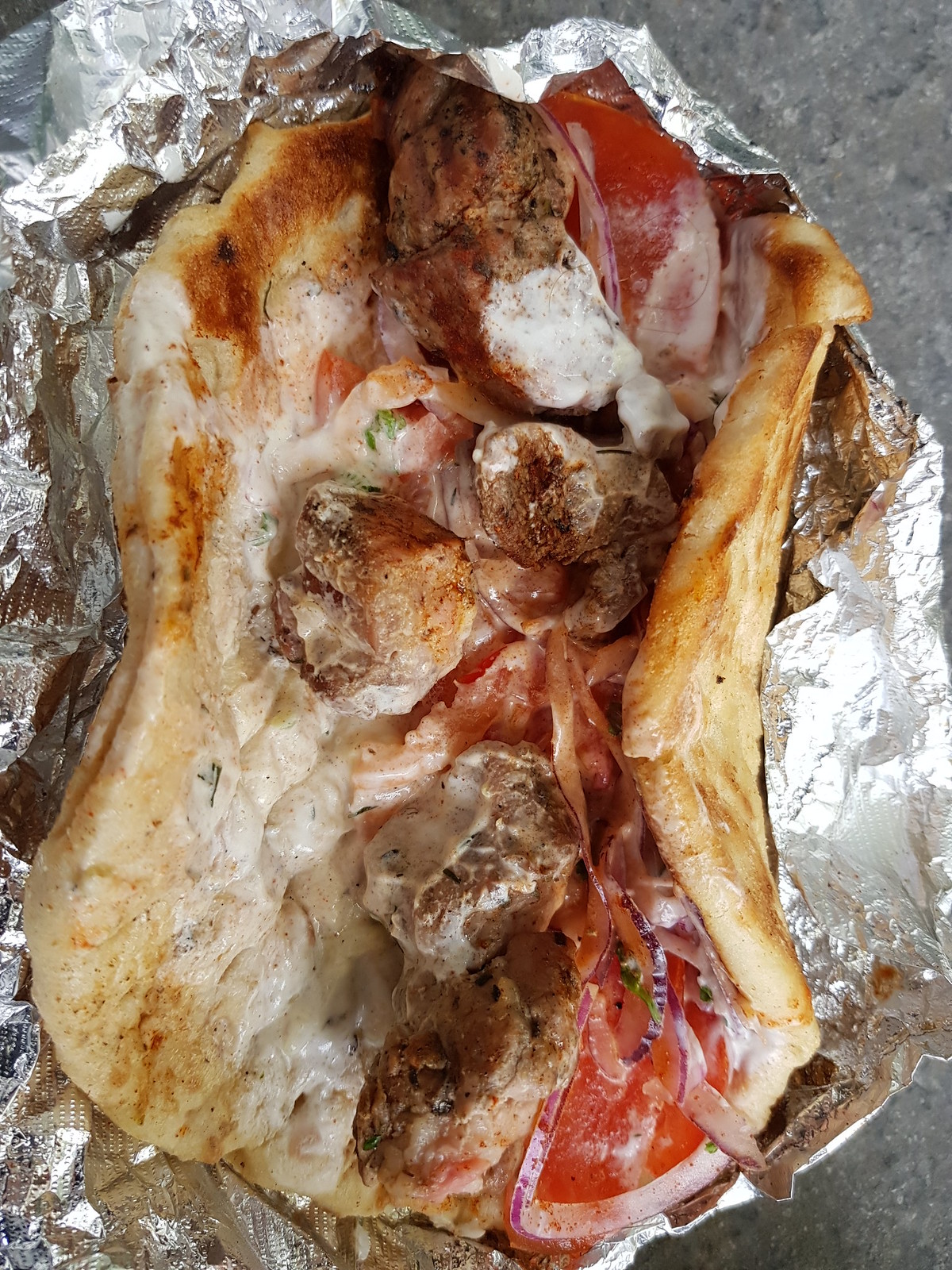This vertically aligned rectangular image displays a delectable food item on top of crinkled foil, which sits upon a gray speckled countertop or table. The focal point of the image is a large piece of meat, most likely a chicken breast, adorned with an abundance of mozzarella cheese, particularly concentrated on the left side. The centerpiece features a variety of toppings: mushrooms, two tomato wedges at the upper and lower right corners, and a slice of red onion also in the lower right corner. Additionally, there appear to be chunks of dark meat, possibly lamb, suggesting a combination of flavors. This visually appetizing dish resembles a Greek gyro wrap with its characteristic ingredients and presentation, reminiscent of classic Mediterranean cuisine. The whole ensemble looks inviting and savory, promising a delectable culinary experience.